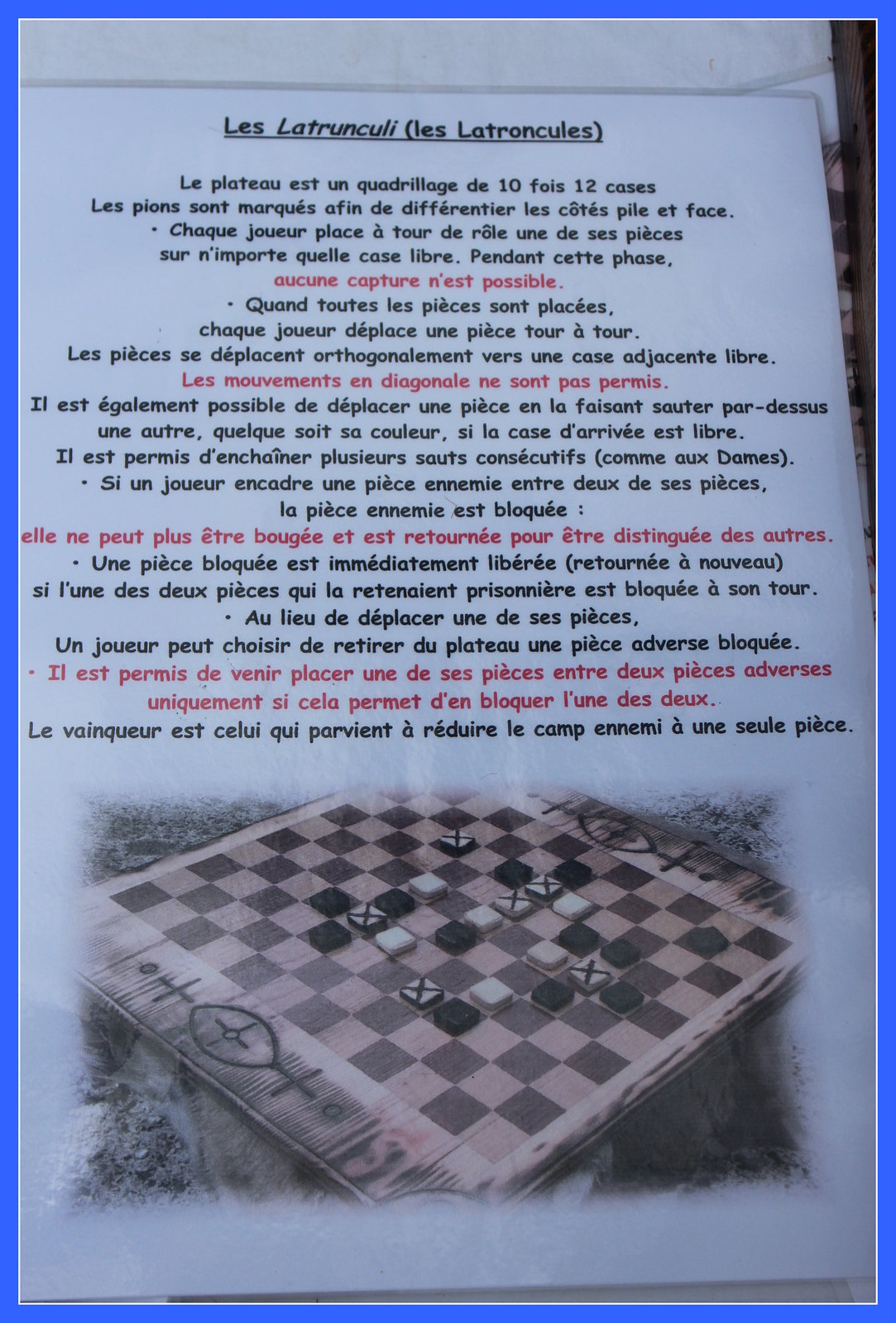This image depicts what appears to be instructions for a French game, titled "Les Lachracelles," at the top. The text is predominantly in black, with some bullet points highlighted in red for emphasis. At the bottom of the image, there is a visual representation of the game board, which combines elements reminiscent of both Go and Chess. The board is larger than a typical chessboard, with square pieces that are black, white, and some white ones marked with X's. Each edge of the board features a symbol resembling a football with a bullseye in the center, flanked by cross signs on either side. The entire image is framed by a blue border, enhancing its visual appeal.